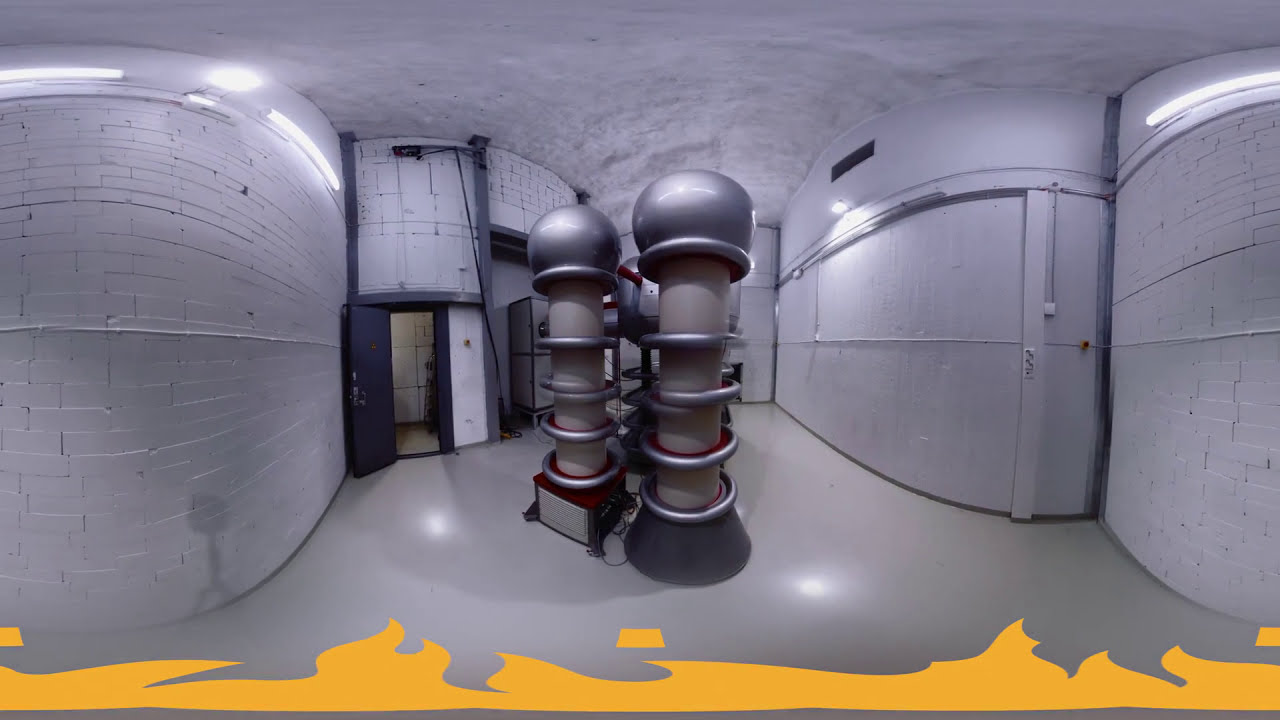This intriguing industrial image, resembling a basement of a power generating facility or an underground science lab, is marked by its peculiar and futuristic vibe. The room is predominantly white, from the floors to the ceiling, with an underlying outline of bricks visible on the walls, giving it a whitish-gray appearance. The floor, though mostly white, features a striking golden-yellow flame pattern, the origin of which is uncertain. At the center of the room stand three silver structures, two distinctly visible, resembling futuristic generators. These structures have thick bases, cylindrical forms with rounded tops akin to mushroom caps, and are encircled by complex tubing. The room is illuminated by fluorescent lights mounted on the ceiling. In the background, there's a blue doorway slightly ajar, adding to the room's enigmatic atmosphere. The image, which has a slight fisheye distortion, evokes a sense of high-tech scientific equipment within an industrial setting.